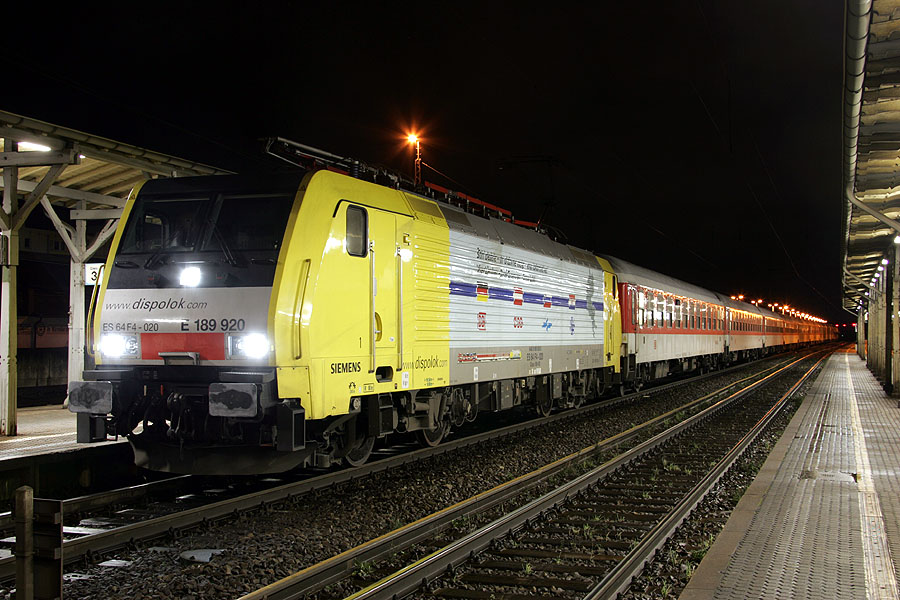The photograph captures a nighttime scene at a train station, with a sleek, aerodynamically built passenger train approaching from the left. The train has a distinctive yellow and gray front, marked with "DispoLock" above the windshield. The lead car is yellow, transitioning into a white body. The trailing cars are distinctive, with the first one being white with a blue stripe and the subsequent cars featuring red sides, gray roofs, and windows. The perspective shows the train on the second track extending into the background, with diminishing perspective towards the upper right. The scene is lit by a single bright light above the train and a red light can be seen near the destination. The platform on the left side of the train is simple and empty, mirroring the deserted right-side depot, with another set of empty tracks closest to the viewer.